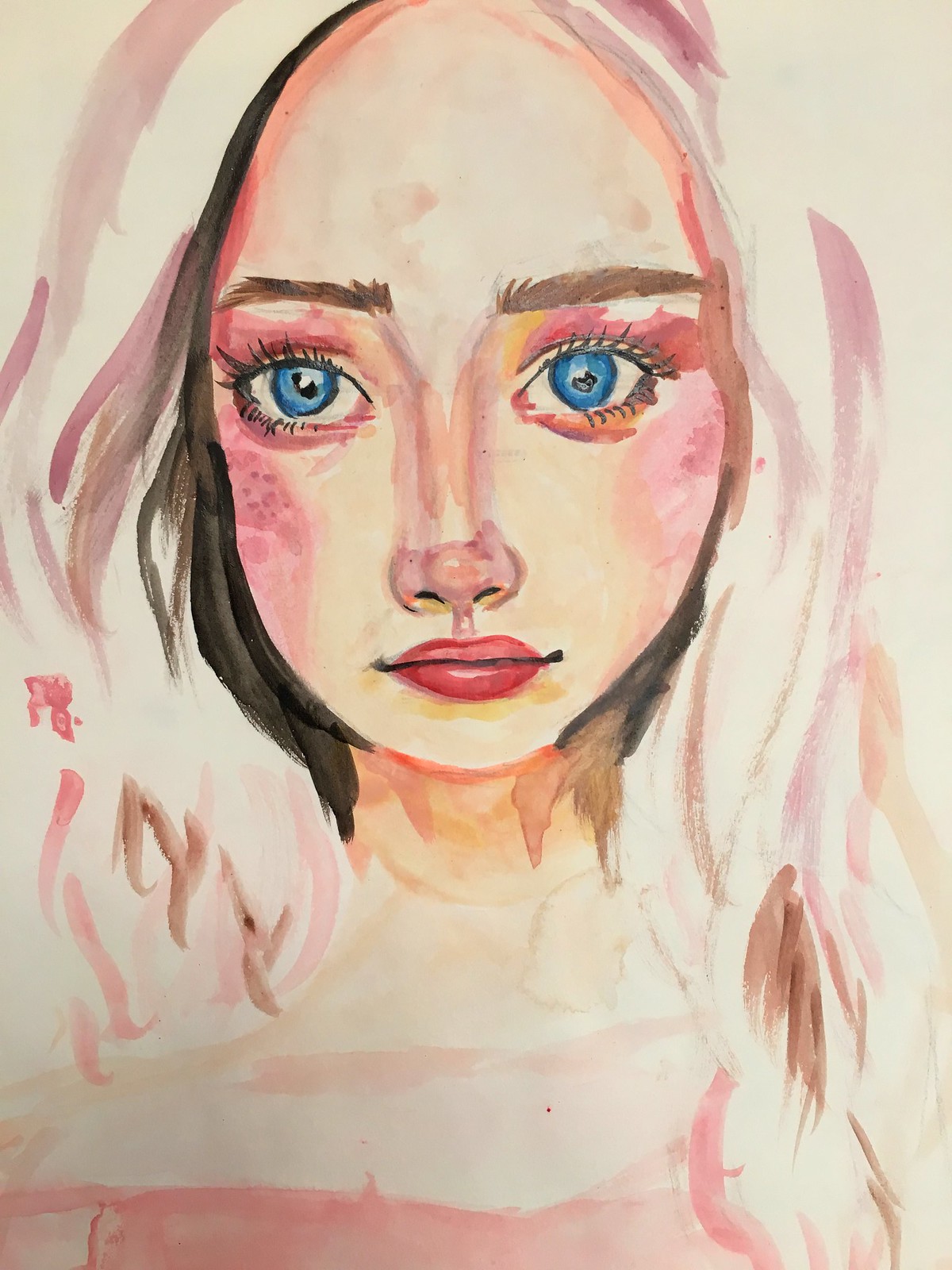This is a highly artistic watercolor drawing or painting of a young woman, seen from the chest upwards. The minimalist portrait features her large, elliptical head that dominates the composition, occupying about half of the image from top to bottom. She has a radiant complexion with tan skin. Her striking facial features include big, expressive blue eyes with a shining glare, highlighted by dark black eyelashes and long horizontal eyebrows, which some descriptions note as black or brown.

Her lips are adorned with red or dark pink lipstick, and she also wears pink eye shadow and eyeliner, accentuating a well-made-up appearance. Her thin nose is positioned close to her mouth, emphasizing her delicate facial structure. 

Her hair is a complex, multi-colored blend of white, black, blonde, light purple, and brown, with pink highlights, adding a vibrant and dynamic quality to the piece. A noticeable detail is a pink bow located towards the left near the bottom of her hair, which further enhances the artistic charm. The hair is depicted as long and wavy, flowing around her face and shoulders.

The woman is dressed in a minimalistic, short sleeveless, pinkish top that ends just around the collarbone area, exposing much of her neck and shoulders. The overall effect is a beautifully rendered, enigmatic portrait that showcases an expert use of color and minimalist detail to capture the essence of the subject.